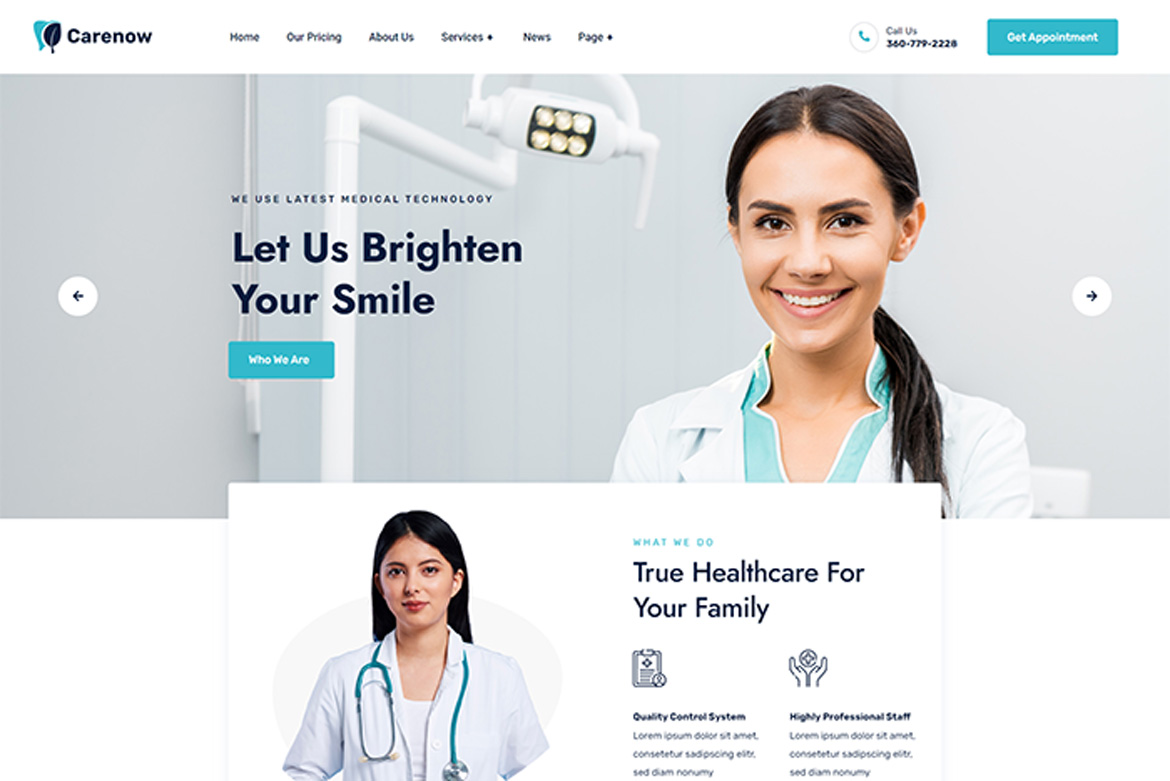A screenshot of the CareNow website prominently features a cheerful woman, with the caption "Let us brighten your smile," suggesting a focus on dental care. The background indicates a dentist's office, reinforcing the dental theme. Below this, another image showcases a different woman wearing a stethoscope, aligning with the message "true health care for your family," indicating a comprehensive range of healthcare services. Two small icons with tiny, unreadable text beneath them accompany this imagery. The website's header includes navigation options: Home, Our Pricing, About Us, Services, News, and an unreadable category. It also provides contact information with a "Call Us" phone number and a "Get Appointment" button, making it easy for visitors to schedule a visit.